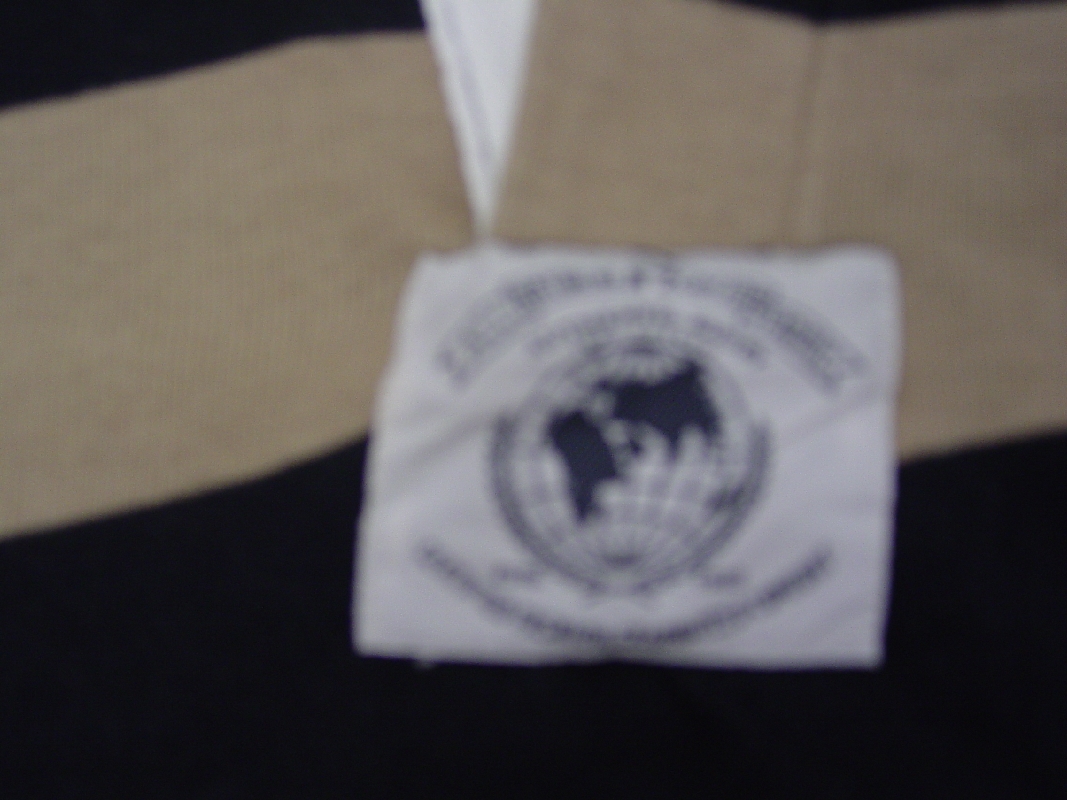In the image, the top left corner features a black section. Directly below this black area, there is a prominent brown stripe that spans across the image. At the center, there is a white square that contains some text, although it is not legible. Inside this white square, there appears to be a depiction of a globe showcasing the African and European continents. The bottom part of the image also displays a rounded black area. The overall composition of the image includes black at the top, followed by a large brown stripe, and then a substantial portion of black fabric at the bottom.